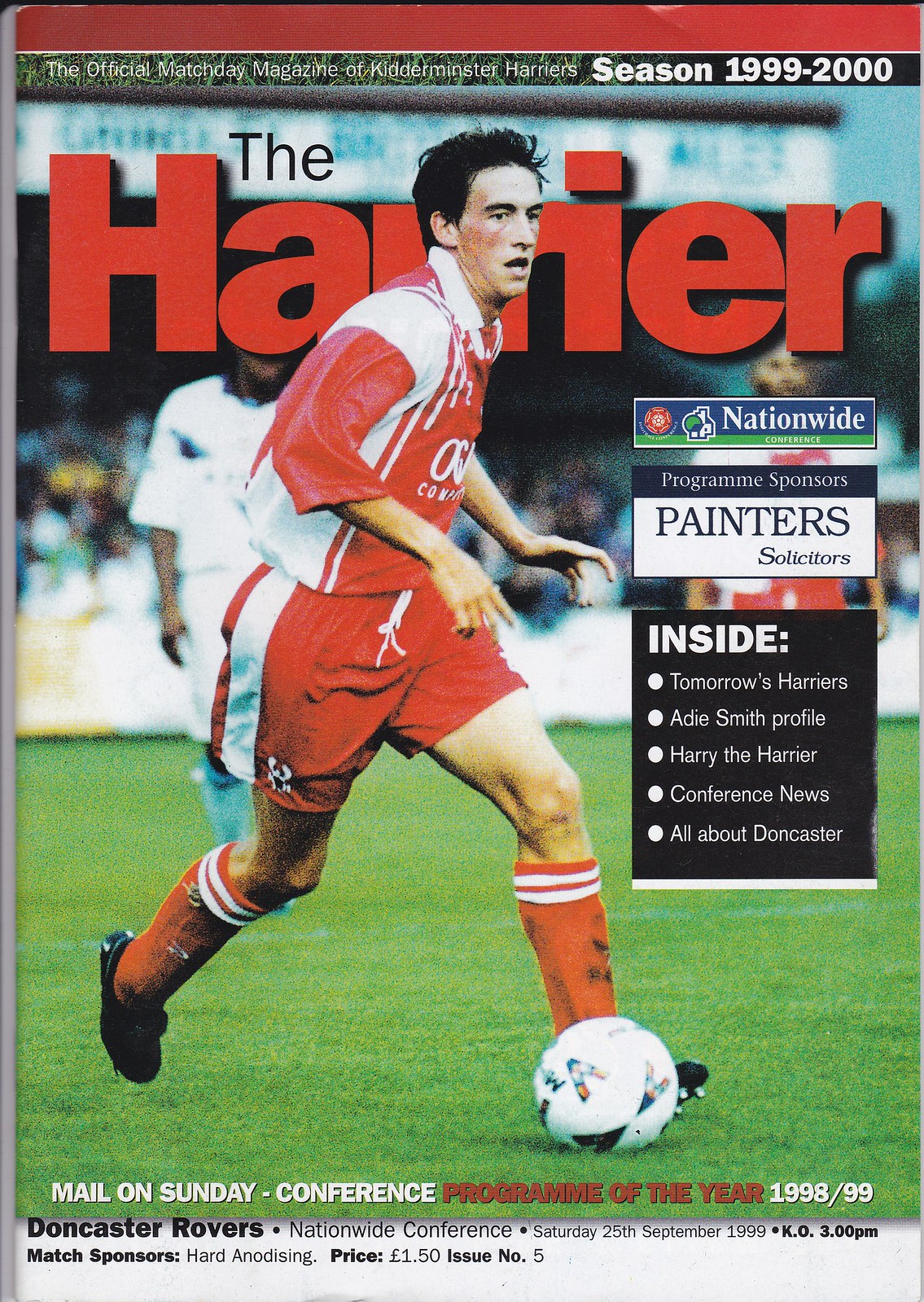The image is an advertisement for the Harrier magazine, featuring a vibrant cover that predominantly showcases a soccer theme. The magazine title, "The Harrier," stands out in bold red text against the background. Central to the cover is a soccer player, identified by his red jersey, red shorts, and red socks with white stripes. He appears to be a white male with dark, short hair, and is shown in a dynamic pose, likely gasping for air as if in mid-action during a game. 

The backdrop behind the player is a green field with some white accents, suggesting a soccer pitch. Additional details highlight the magazine’s significance; it is labeled as "The Official Match Day Magazine of the Something Harriers," for the season 1999-2000. Above and below the player, there is text indicating that it was awarded the "Mail on Sunday Conference Program of the Year" for 1998-1999. 

Further information includes a mention of "Doncaster Rovers" and a pricing detail, stating the magazine costs £3.00 or $1.50 and is labeled as issue number 5. Various other text elements in white and black provide insights into what can be found inside the issue, including "Nationwide Painter Selectors Inside" and "Tomorrow's Harriers." This cover not only highlights the sport but also offers a historical glimpse into the specific season it documents.